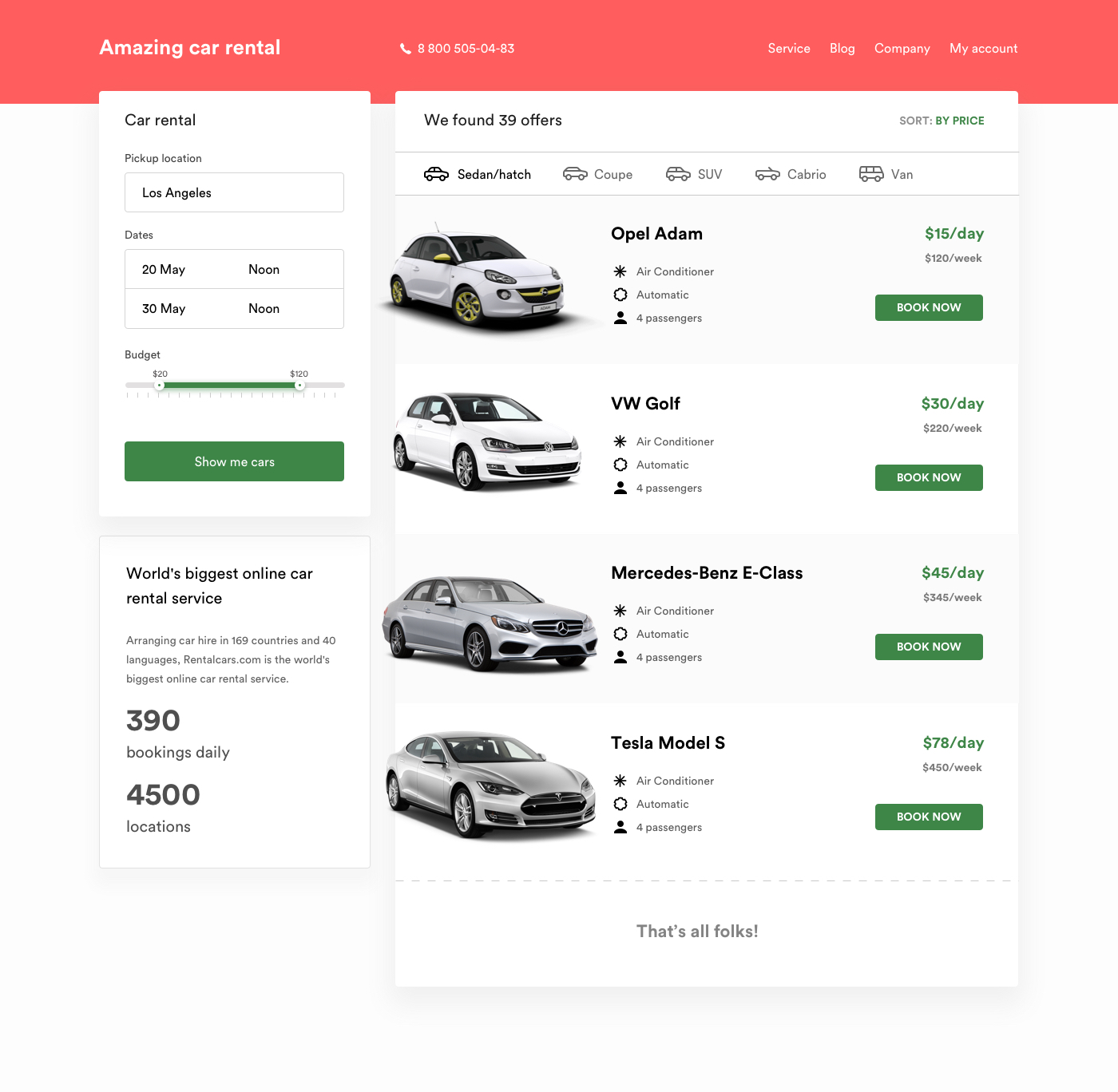A detailed screenshot of the Amazing Car Rental website is presented. The image features a prominent rectangular pink header displaying the site's name, “Amazing Car Rental,” where "Amazing" is capitalized, and "Car Rental" is in lowercase. Adjacent to the site’s name is a contact number: 1-800-505-0483. Next to this, there are four navigation categories: "Service," "Blog," "Company," and "My Account," all encapsulated within the pink header.

Below the header, on the left side, there is a section dedicated to car rentals titled "Car Rental" with a green button labeled "Show Me Cars," featuring white text. Directly beneath this, a messaging banner touts, "World's Biggest Online Car Rental Service," accompanied by statistics on daily bookings and location availability.

On the right side, the main content reveals details about the search results for car rental offers. Users can sort these results by price. The categories include:
- Sedan/Hatch
- Coupe
- SUV
- Cabrio
- Van

Further down are the specific listings, each with a car model, daily rental rate, and a "Book Now" button:
1. Obel Atom - $15 per day
2. VW Golf - $30 per day
3. Mercedes Benz E-Class - $45 per day
4. Tesla Model S - $75 per day

At the bottom of the page is a playful sign-off: "That's all folks."